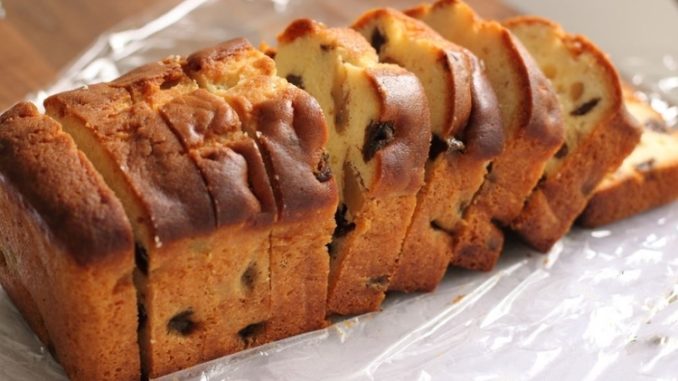The image is a high-quality, side-angled photo of a handmade, square loaf of bread, baked to a golden deliciousness. The loaf, which occupies the majority of the picture and is laid out diagonally on a sheet of shiny cellophane, is predominantly light-colored with noticeable inclusions of raisins and possibly swirls of cinnamon, suggesting it might be a raisin cinnamon swirl bread. It is precisely sliced into 9 even slices, each about half to one inch thick, with no pieces missing or displaced. The slices are arranged in such a way that the loaf remains intact and inviting, ready to be grabbed and eaten. The bread appears freshly made, either homemade or recently purchased, with definitive crumb evidence on the plastic sheet. There are no other objects or text present in the photo, and nothing is spread on the bread, indicating its flavor is meant to be enjoyed as is. This is not the type of bread for sandwiches but rather a flavored specialty bread perfect for standalone enjoyment.